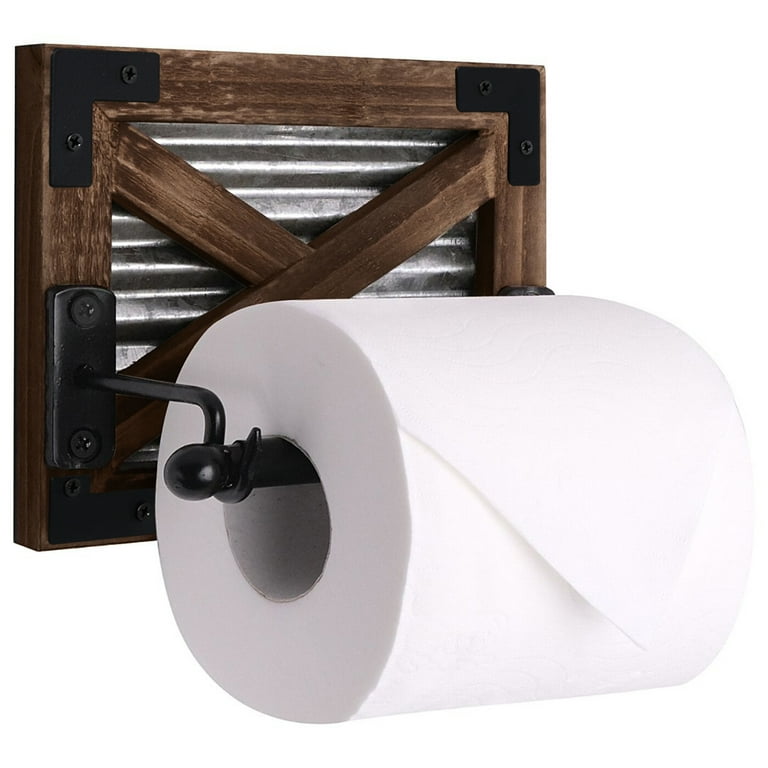The image shows a beautifully arranged roll of white, quilted toilet paper hanging neatly from a uniquely designed toilet paper holder. The toilet paper is meticulously folded into a triangle at the start, giving it an untouched and pristine appearance. The holder features a distinctive and stylish design: a square wooden frame with a rich dark brown finish, intersected by two diagonally crossing wooden beams forming an X-shape. This wooden frame is mounted to a backdrop of sheet metal that has a silver hue, adding a contrasting industrial touch to the rustic look. The toilet paper is suspended on a sleek black rod, which extends from sturdy black metal hooks. These hooks are secured to the wooden frame by visible black screws, adding to the robust aesthetic. Additional black plates reinforce the corners of the holder, completing the elegant and functional design.